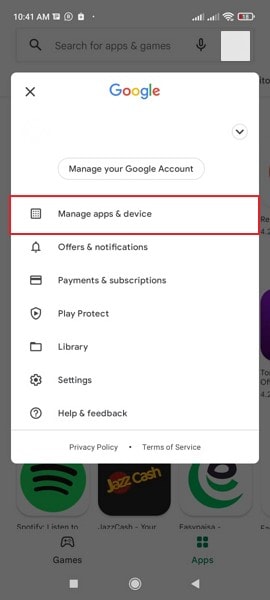The top left corner of the image displays the time as 10:41 a.m. On the right side, the battery life indicator shows 12%. The background area is gray, making visibility slightly challenging. Near the top, there's an icon of a magnifying glass followed by a search bar. Below this, an 'X' symbol is present. The Google logo is prominently featured, with the letters "G" in blue, "o" in red, another "o" in yellow, "g" in blue, "l" in green, and "e" in red.

Approximately two inches below the Google logo, there's an option to manage your Google Account. Positioned below this, a highlighted option with red borders reads "Manage apps and device." Additional options listed include "Offers and notifications", with a credit card icon beside it; "Payments and subscriptions", "Play Protect" represented by a small flag inside a circle, "Library" marked by a book icon, "Settings" signified by what appears to be a clock with a black square in the center, and "Help and feedback" indicated by a question mark inside a circle.

At the bottom of the image, there's a section dedicated to various apps and games available for installation on your phone.